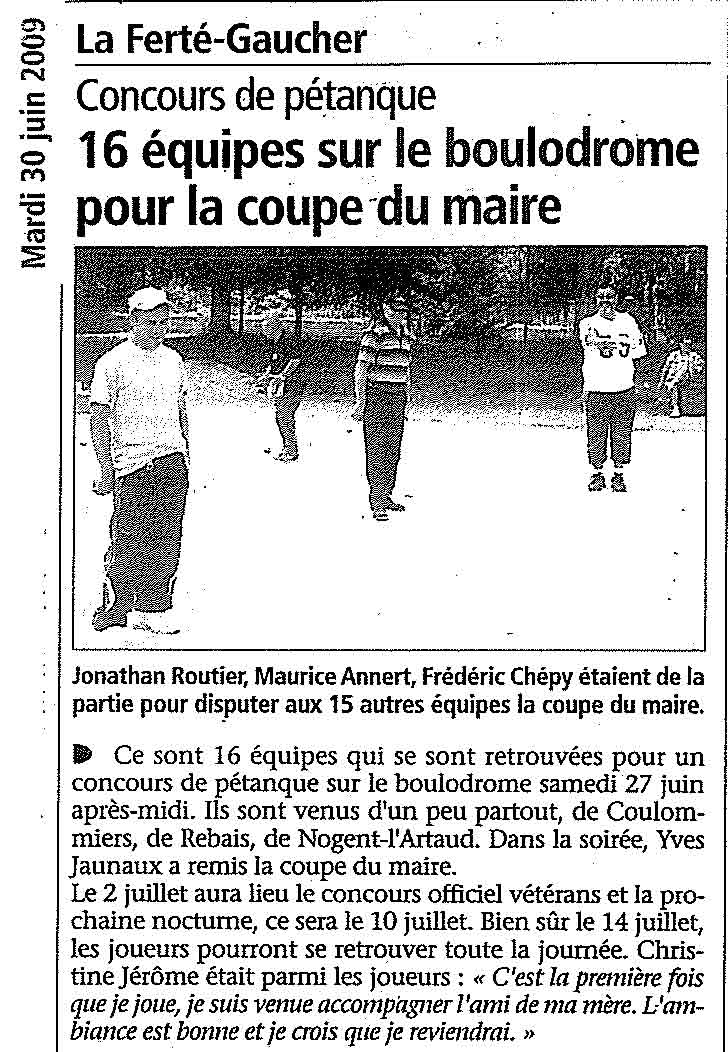The black and white newspaper clipping, dated "Mardi 30 June 2009," features an article in French describing a Pétanque competition held in La Ferté Gaucher. The headline reads, “Concours de Pétanque: 16 équipes sur le boulodrome de Rampolla Côte de Mer,” highlighting the participation of 16 teams. The image within the article shows four men—Jonathan, Maurice, and Frederic among them—standing in a field with trees visible in the background, all looking at the camera while dressed in pants and t-shirts. To the right, a fifth individual is sitting, also looking towards the camera. The photograph includes annotations providing the names of the participants and details about their involvement. Below the image, two paragraphs of text in French further elaborate on the event and its proceedings. The article captures a moment from the competition, visually and textually documenting the day’s activities.